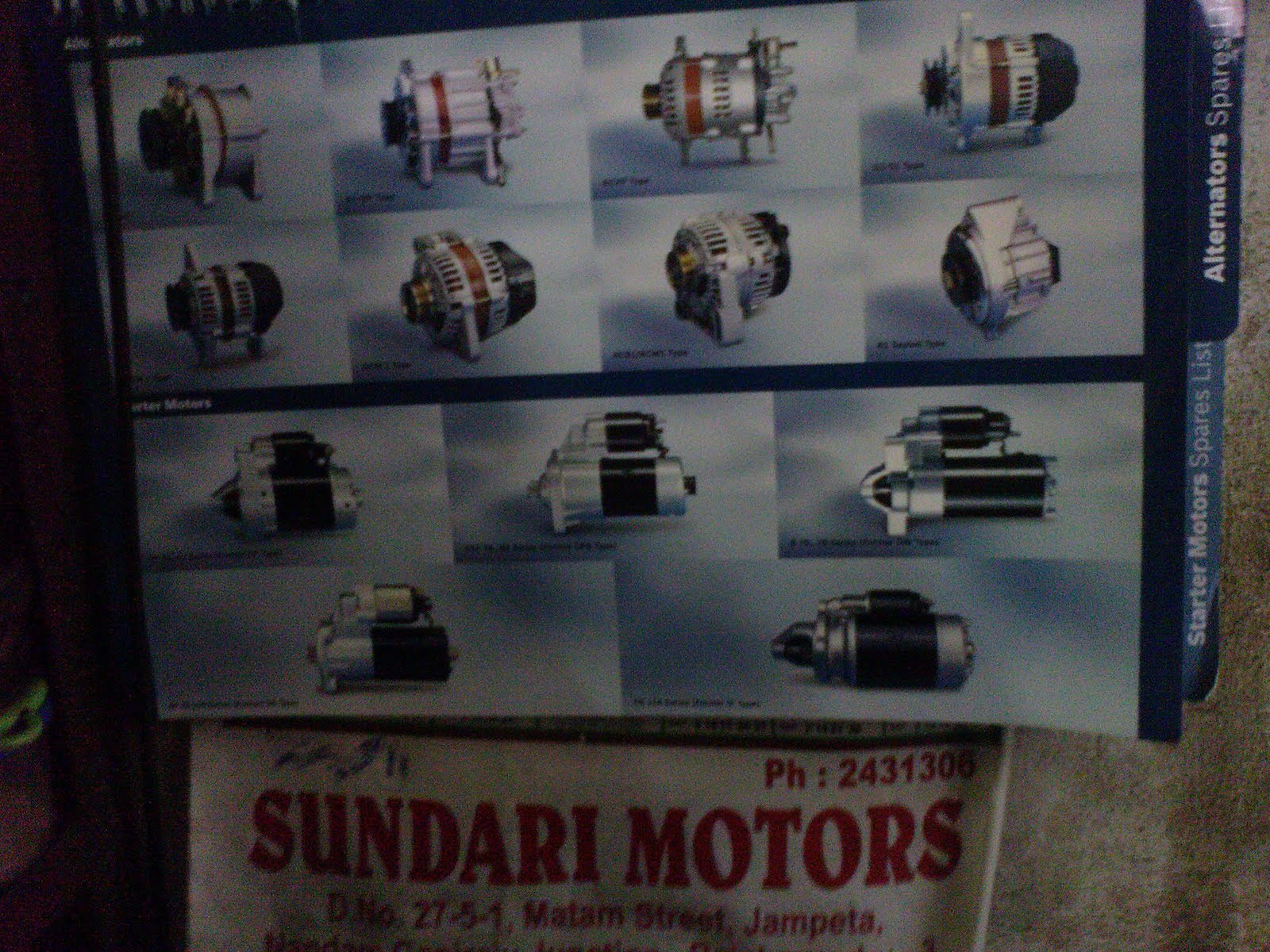This image depicts a detailed catalog page showcasing various alternators and starter motors, primarily for automotive use. The catalog, set against a light blue sheet of paper, is structured with an upper section containing two rows of five alternators each, followed by a lower section with a row of three and a bottom row of two alternators. These machinery parts are predominantly black and silver, with five or six featuring a distinctive red strip around them. On the right side of the catalog, small tabs distinguish the sections, with "Alternators Spares" at the top and "Starter Motors Spares List" at the bottom. Below the catalog is a white piece of paper with red lettering, detailing an advertisement for Sundari Motors, including their address at DNO 2751 Matam Street, Jampeta, and phone number PH: 2431306. The catalog and the advertisement are affixed to what appears to be a concrete wall, captured in a photorealistic style, providing a clear and informative visual representation of the items available from Sundari Motors, based somewhere in India.